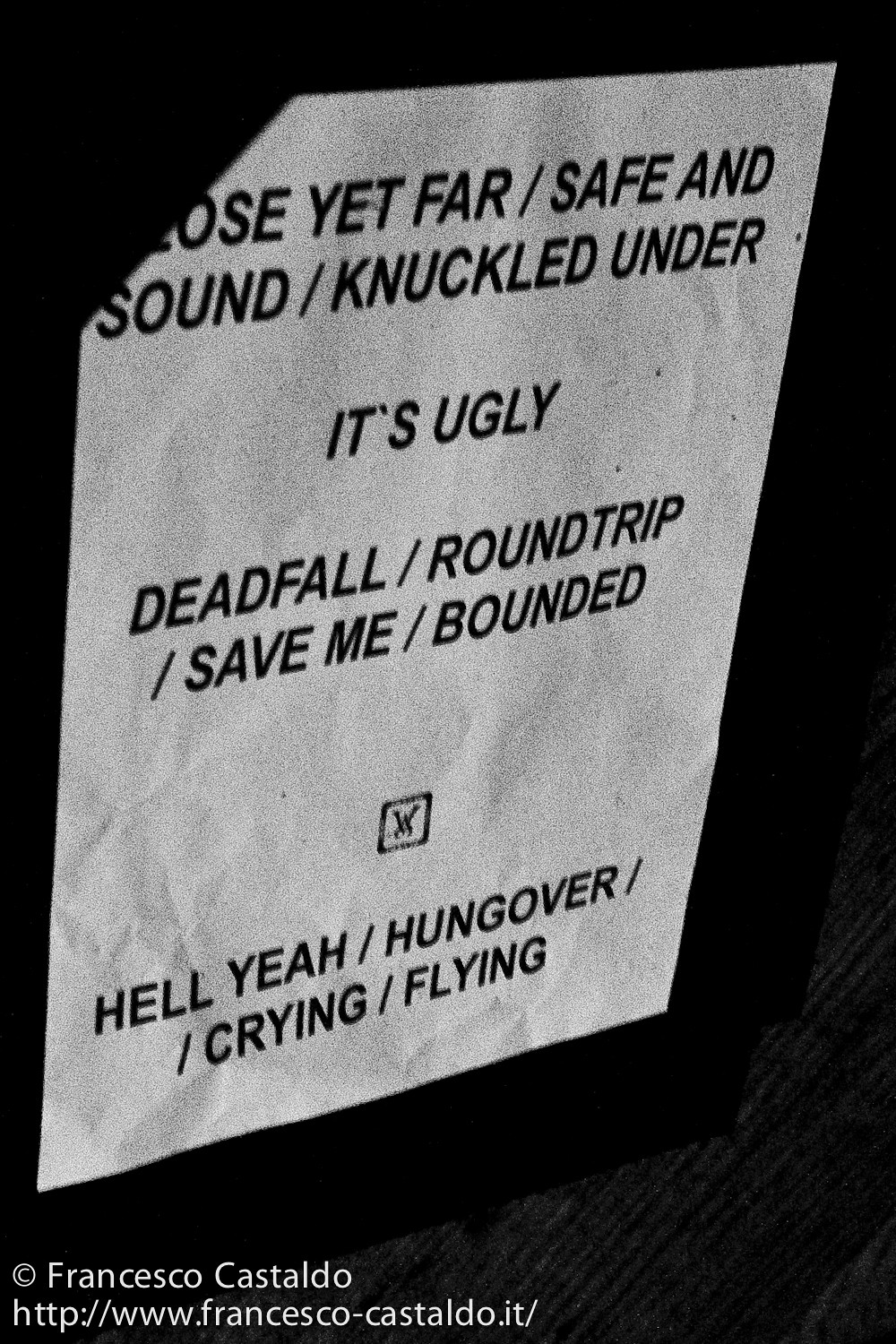In the center of the image is a slightly wrinkled, off-white piece of paper with black text, positioned against a completely black background. The paper seems aged, possibly representing an artistic or thematic concept. The text on the paper appears to be a series of phrases, possibly song titles or poetic lines, organized into distinct sections. 

At the top of the paper, the text reads: "Close yet far / Safe and sound / Knuckled under," followed by a large gap. Below this, centrally aligned, is the phrase: "It's ugly." Another gap follows, leading to: "Deadfall / Round trip / Save me / Bounded." Beneath this, there is a logo that resembles a square with an intersecting V and an upside-down U meeting at their bottoms. The bottom section of the paper reads: "Hell yeah / Hungover / Crying / Flying."

In the lower-left corner, the paper credits Francesco Castaldo, followed by his website URL. The overall composition, with its stark contrasts and lined arrangement, gives the impression of an advertisement or an artistic presentation of lyrical content.